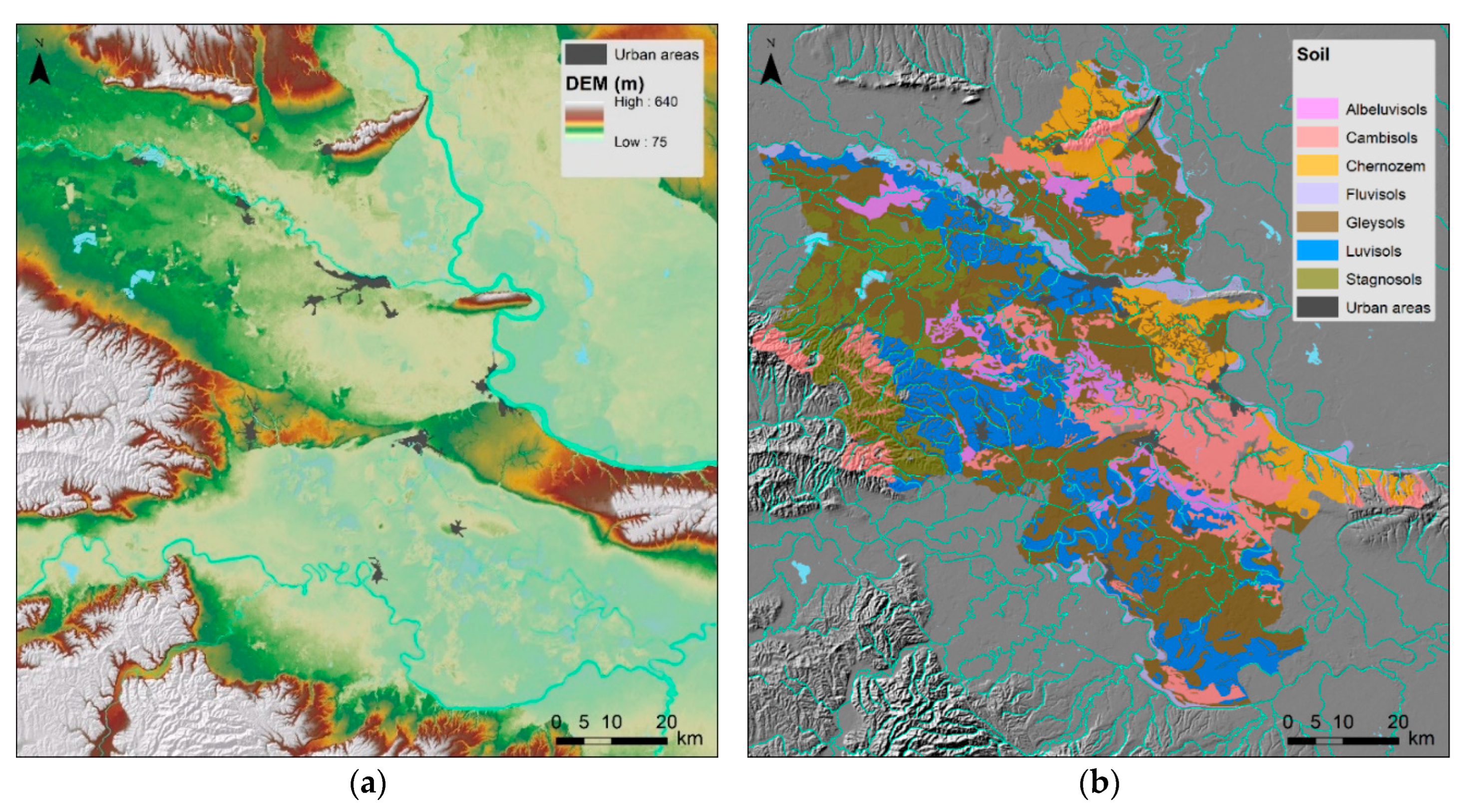This image features two maps labeled "Map A" on the left and "Map B" on the right, each representing the same geographic region but displaying different types of information. 

**Map A**, predominantly green with patches of red, white, and black, includes blue lines indicating water bodies. The legend at the top right designates dark gray areas as urban zones. Additionally, it labels various density elevations, marked as D-E-M (M), with values ranging from a high of 643 to a low of 75. In the bottom right, a scale denotes distances of 0, 5, 10, and 20 kilometers, with the focus of interest between the 5 and 10 km marks.

**Map B**, characterized by a grey background with accents of pink, green, blue, yellow, orange, and brown, has a top right legend that categorizes soil types. This legend reads: cyan for Albuviosols, pink for Cambisols, yellow for Chernozems, pastel purple for Fluvisols, brown for Gleysols, blue for Luvisols, green for Stagnosols, and dark gray for urban areas. The distance scale similarly shows 0, 5, 10, and 20 kilometers, with a key focus between the 5 and 10 km intervals.